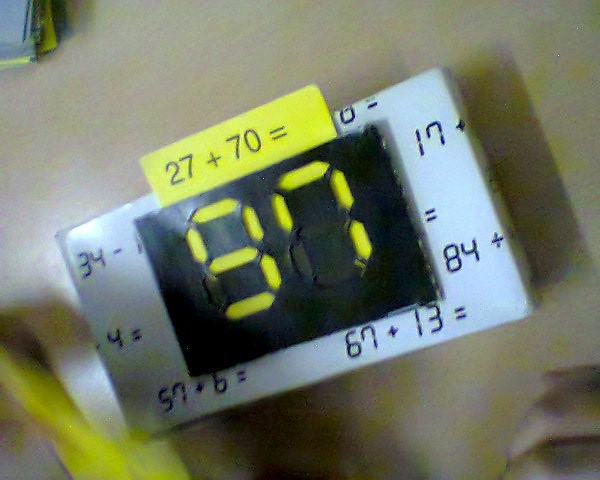The image depicts a slightly blurred, homemade or handcrafted calculator-like device photographed at a slanted angle from bottom left to top right, on a tan-colored tabletop. The central section of the device is a black rectangle displaying digital-like yellow numbers, prominently showing '97'. Encircling this digital readout is a white frame filled with mathematical equations and symbols, such as "67 + 13," "57 + 6 =", and "34 -". Positioned above the digital screen is a yellow strip of paper with black text stating "27 + 70 =." Several human fingers are visible in the lower right corner of the image, and a pile of paper can be seen in the top-left corner.